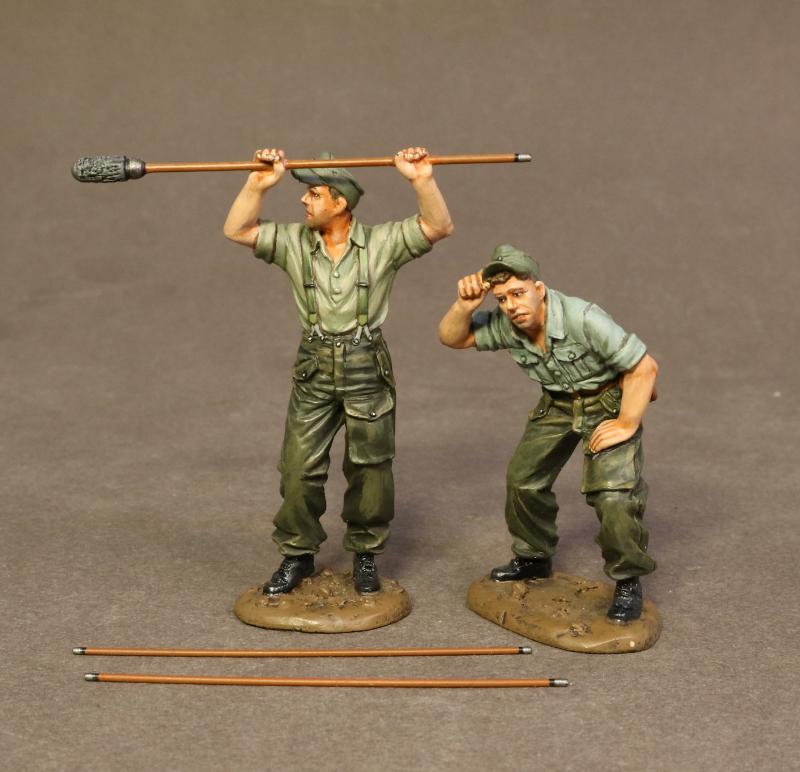The image features two well-detailed toy figures, potentially made of metal or plastic, and seemingly representing soldiers, likely German given their caps. Both figures are dressed in light green shirts - one with sleeves rolled up above the elbows - and matching olive-green pants. One figure wears suspenders while the other does not. They are equipped with black army boots and green caps, typical of military attire. 

The figure on the left stands firmly, grasping a long rod with a swab-like end above his head, suggestive of an artillery tool used for swabbing out barrels. He appears muscular, his attire resembling heavy work clothes, hinting at laborious tasks. The figure on the right is slightly bent over, his right arm raised to his head as if shielding his ear, the other resting on his knee, simulating a stance of intense focus or reaction to a loud noise.

Below them lie two brown rods with silver tips, likely representing tools related to their artillery work. The background is a simple brown, enhancing the focus on the figures which measure approximately six to seven inches in height, adding to the impression of miniature soldiers on duty.